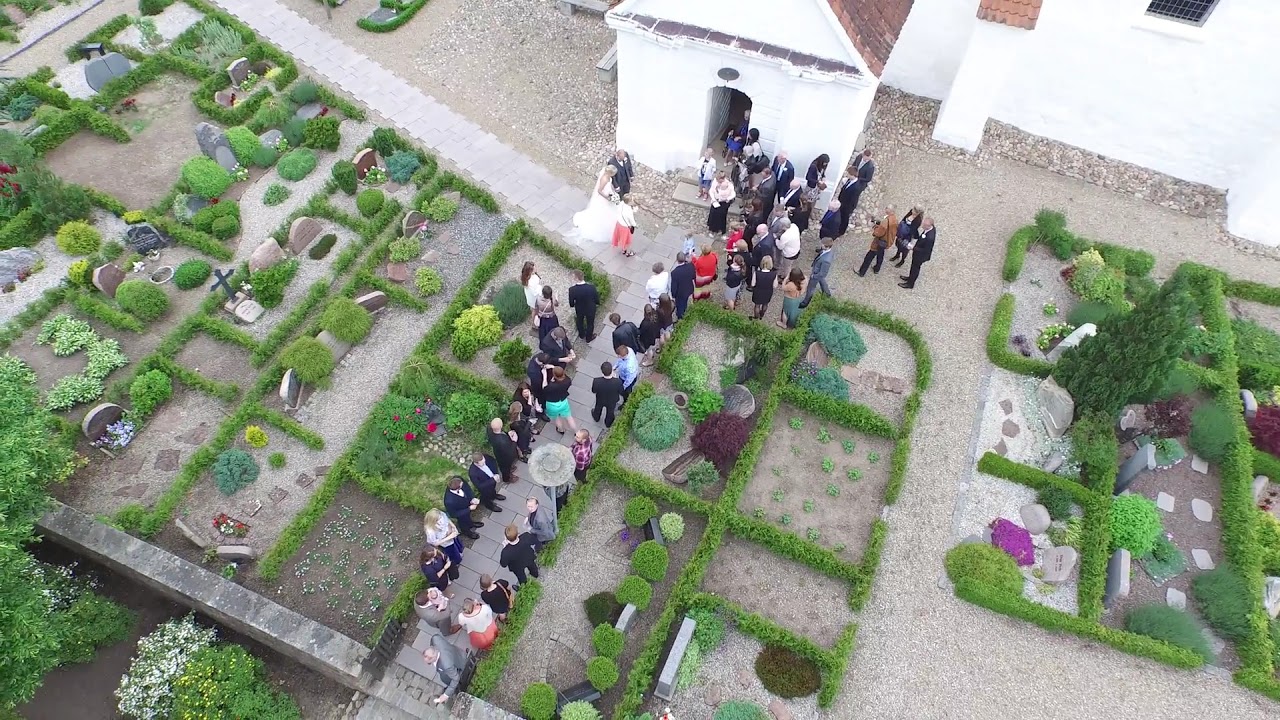This landscape-oriented color photograph captures an overhead view of a wedding procession taking place outside a small white chapel with a red-tiled roof and narrow arch doorway, situated in the upper center of the image. The bride, wearing an elaborate white gown with flowers in her hair and holding a bouquet, stands beside the groom in a black suit on a cobbled stone path to the left of the chapel doorway. Guests dressed in subdued wedding attire, some holding parasols to shield themselves from the sun, line both sides of the walkway, creating a corridor for the couple. The scene unfolds in a vibrant garden-like cemetery filled with lush green bushes, colorful flowers, and arranged grave sites marked by headstones and crosses, each bordered by neat green hedges. The gray gravel and cobblestone pathways, coupled with the greenery and the serene ritual taking place, evoke a poignant and picturesque atmosphere.